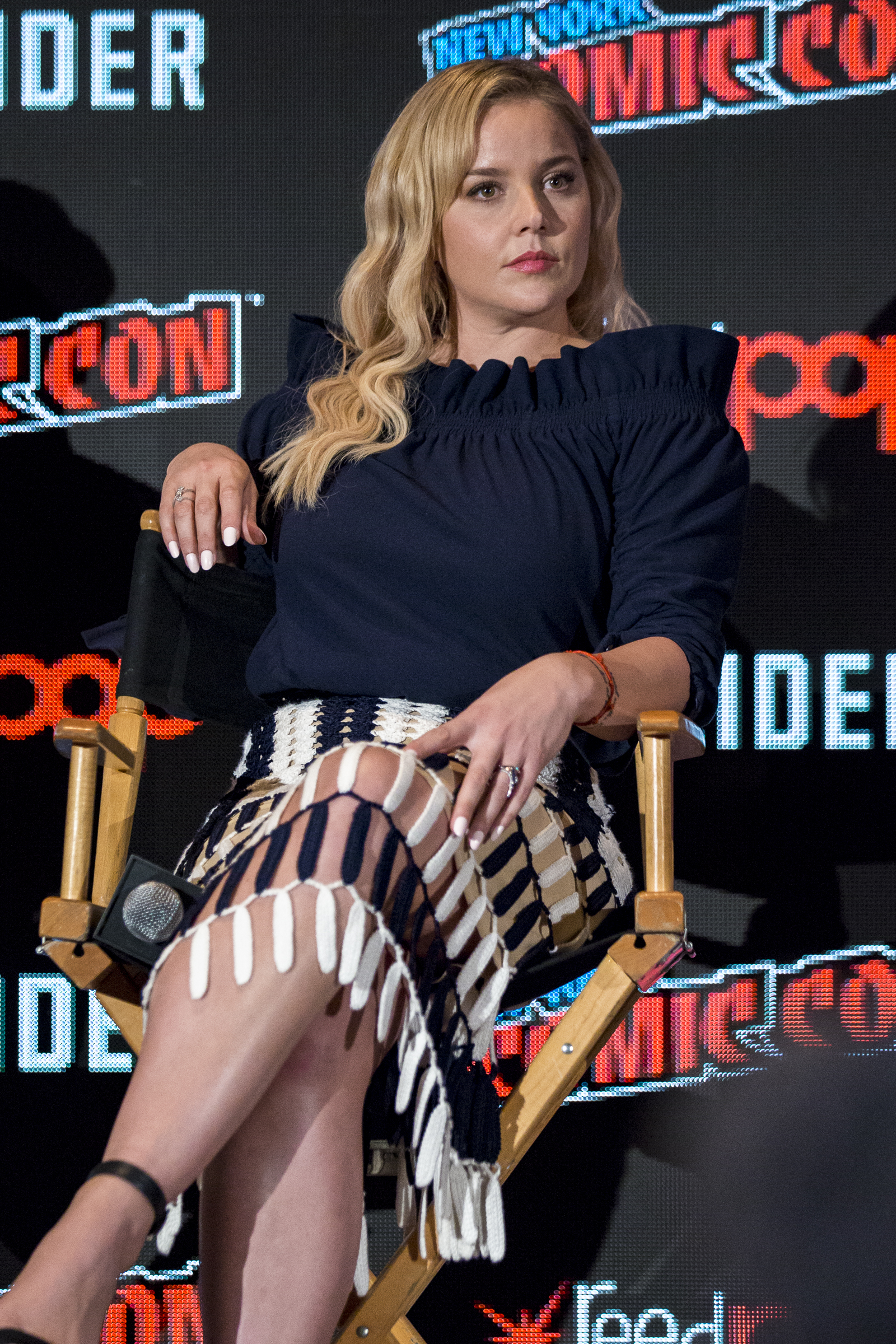In this photograph, a woman, likely in her late 20s to early 30s with long, wavy blonde hair, is seated on a wooden director's chair on a stage. Her attire is both elegant and distinctive: she wears a dark blue, frilly top and a partly see-through skirt with alternating black and white beaded panels. She has white nail polish, light red lipstick, and looks focused, adding to her poised and perhaps "no-nonsense" demeanor. The chair has a black cloth backing, and she holds a microphone with a black square base on the seat next to her legs. Both of her arms rest on the dual-level armrests of the chair. Positioned in front of a large, mostly obscured banner with "Comic Con" partially visible, her setting suggests she is an actress participating in a comic convention.